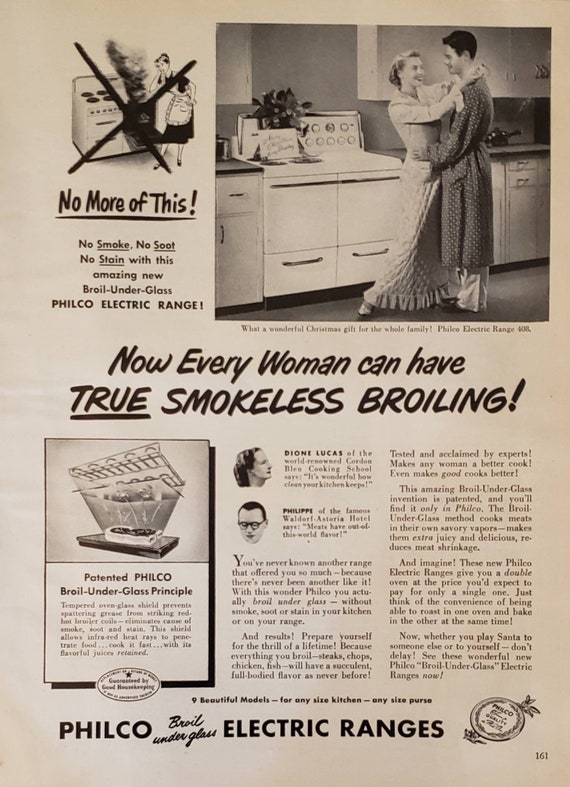The image represents an aged, sepia-toned advertisement from a vintage magazine, appearing to be a page from a newspaper or promotional booklet with the page number 161. The ad showcases the Philco electric stove, emphasizing its innovative "broil under glass" technology. The main text incorporates bold headings such as "No more of this! No smoke, no soot, no stain," promoting the revolutionary smokeless broiling feature. The page features multiple images, including a large oven emitting smoke and a woman in an apron looking distressed, as well as a romantic scene of a couple in a kitchen, with the man in pajamas and the woman in a white gown, surrounded by kitchen cabinets and utensils. Highlights include endorsements from experts, emphasizing the cleanliness and exceptional taste achieved with the Philco electric range. The advertisement also stresses the convenience of a dual-oven setup, allowing simultaneous roasting and baking. At the bottom, the ad mentions "nine beautiful models for any size kitchen, any size purse," reinforcing its appeal as a perfect Christmas gift for the family. The brand name "Philco" and the product's unique features are displayed prominently, alongside assurances of quality and satisfaction.